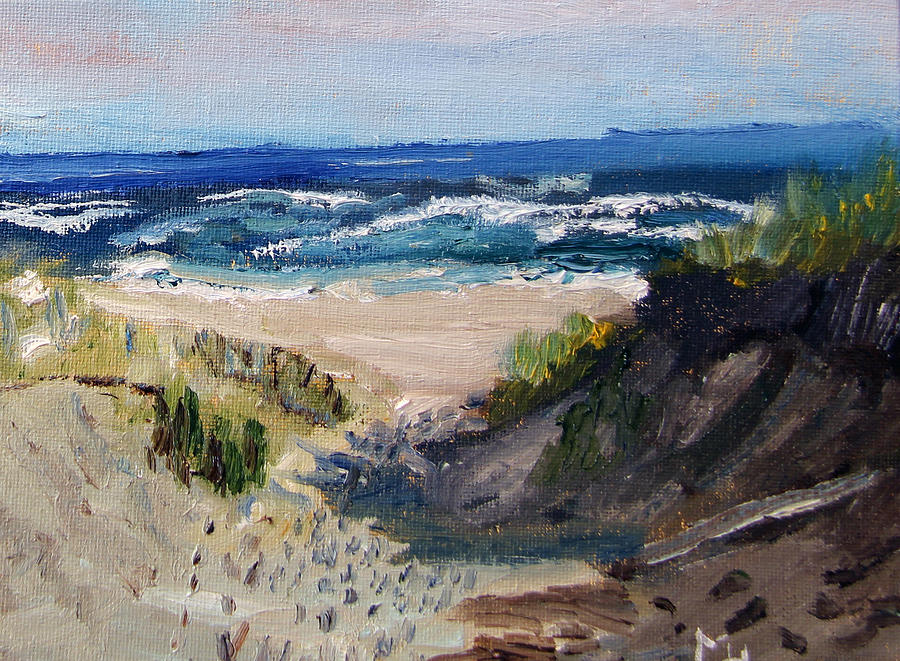This painting depicts a coastal scene characterized by its expressive and somewhat rough brushwork, prominently featuring red strokes. The upper portion of the canvas illustrates the ocean, rendered in varying shades of blue and white to capture the dynamic texture of crashing waves against the shore. The waves create a frothy white effect as they break, enhancing the overall sense of movement in the piece.

The foreground comprises a sandy beach, painted in a warm tan hue, conveying the natural color of the sand. On the right side of the painting, there is a rugged rocky hillside, adorned with patches of green vegetation that hint at grass clinging to the stony terrain. 

The left side of the painting showcases a sandy dune, modeled in a darker tan color, suggesting the accumulation of sand pushed up by the relentless waves. This sand hill is also dotted with grass, indicating a less disturbed area where vegetation manages to thrive. Overall, the painting captures the serene yet dynamic essence of a coastal landscape with its interplay of elements and textures.